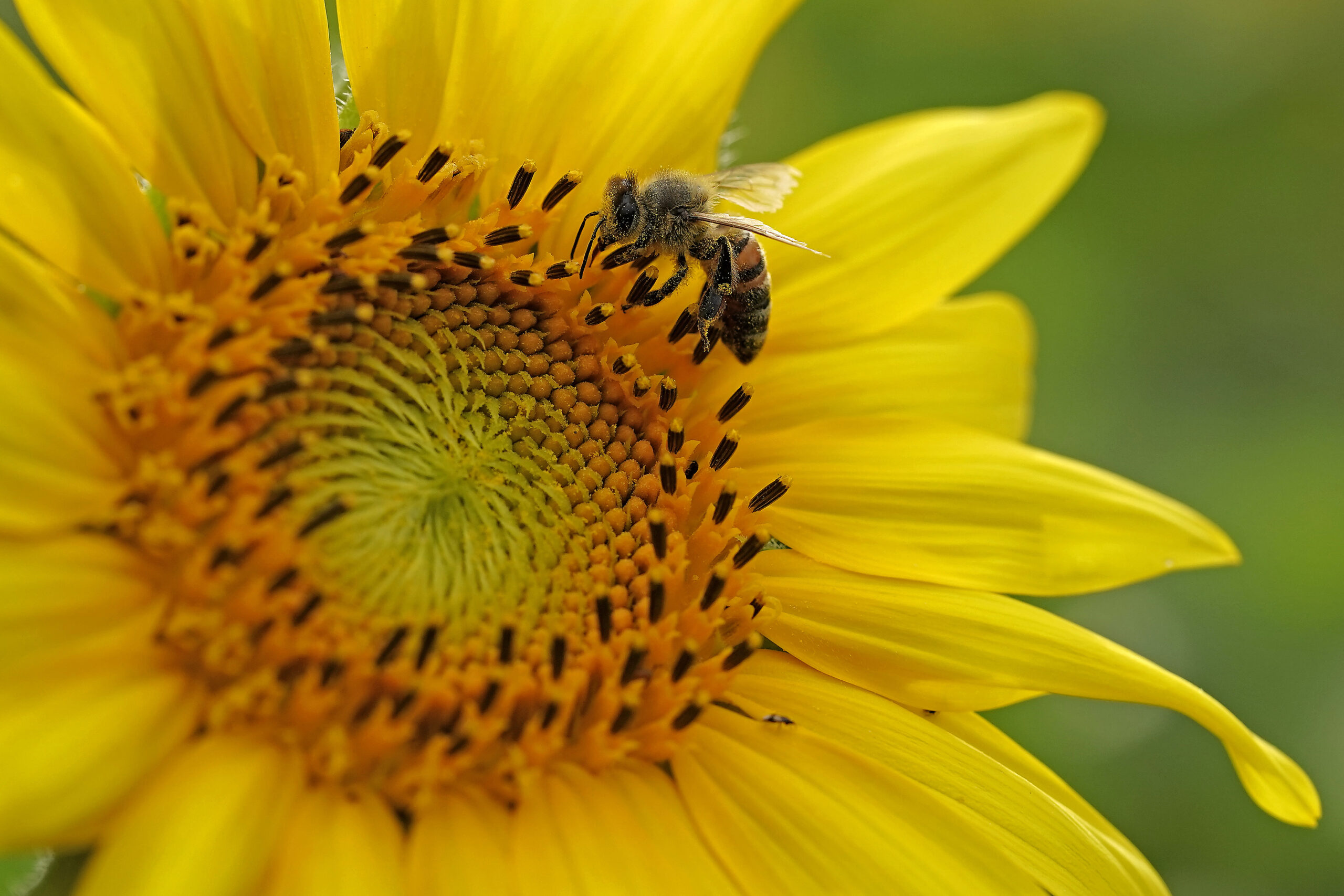The image is a close-up, professional photograph of a vibrant yellow flower, likely a sunflower or a daisy. The flower occupies most of the frame, particularly the left side and extending towards the right. The petals are long, tapered, and velvety, with vertical lines running through them. The center of the flower is a mix of colors, from a dark orange core to a lighter, golden yellow with tiny, bumpy black bits and small, tubular shapes protruding.

A honey bee, identifiable by its fuzzy head and striped yellow and black abdomen, is prominently featured in the image. The bee is engaged in collecting pollen, with its black-tipped, yellow antennae dipping towards the flower’s center. Its wings are clear and visible, adding to the intricate details captured by the close shot.

The background is an out-of-focus blur of various shades of green, providing contrast that emphasizes the sharp, vivid details of the flower and the bee. The image showcases expert use of aperture to create this depth of field, making the primary subjects—the flower and the bee—stand out clearly against the blurred background.